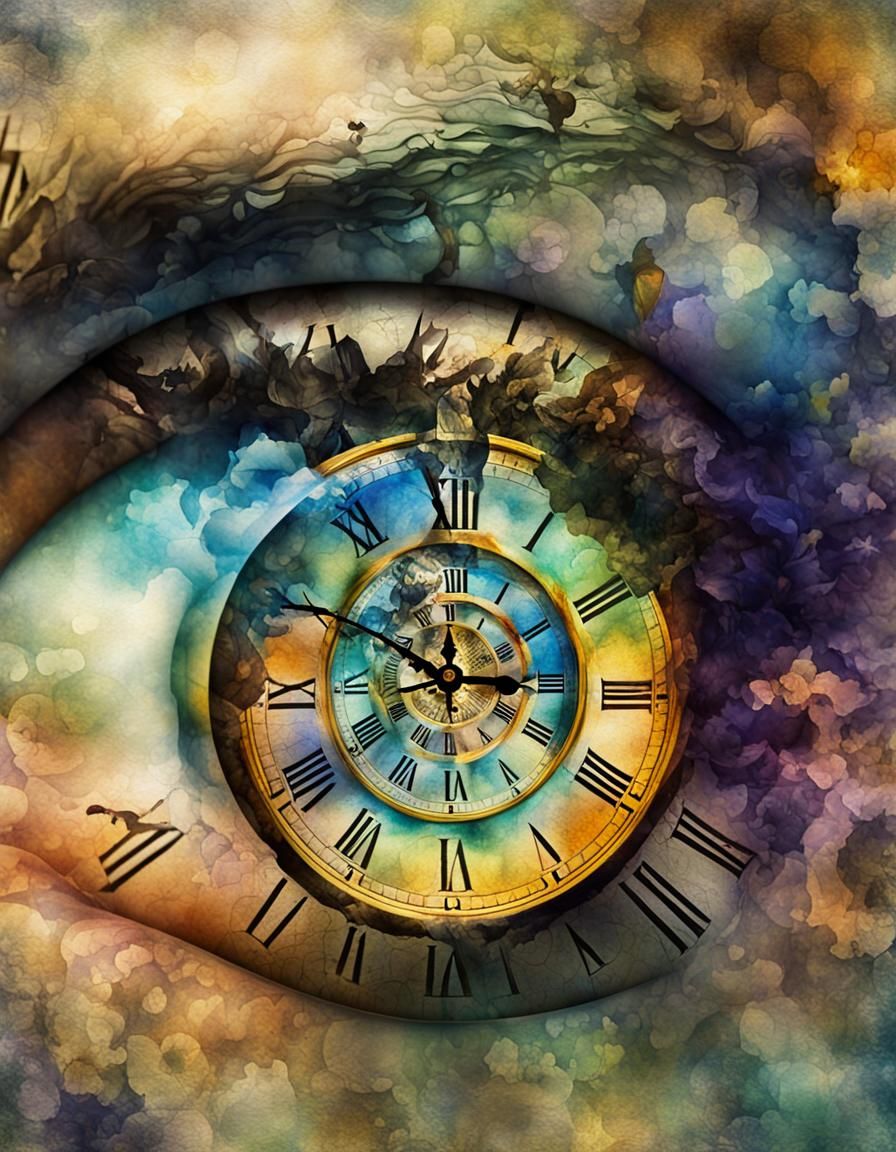This abstract artwork appears to be either a painting or a computer-generated piece that zooms in on what seems to be a woman's eye. The eye is depicted with a striking level of detail that includes a visible eyebrow right above it. Uniquely, the pupil of the eye contains a spiral of multiple clocks set within each other, forming a mesmerizing, almost surreal effect.

The clocks display various numbers and hands in layers, creating an intricate, complex pattern at the center of the eye. Each clock frame appears to be rendered in gold or bronze. The entire image is awash in a blend of soft yet bold pastel colors, including blues, greens, yellows, oranges, pinks, and purples. These colors seamlessly mix and blend with one another in a watercolor-like style, extending across the eyelid and onto the eyelashes.

The overall effect is a captivating blend of elements that highlight both the eye and the clocks, making it a compelling depiction of the convergence of time and vision.